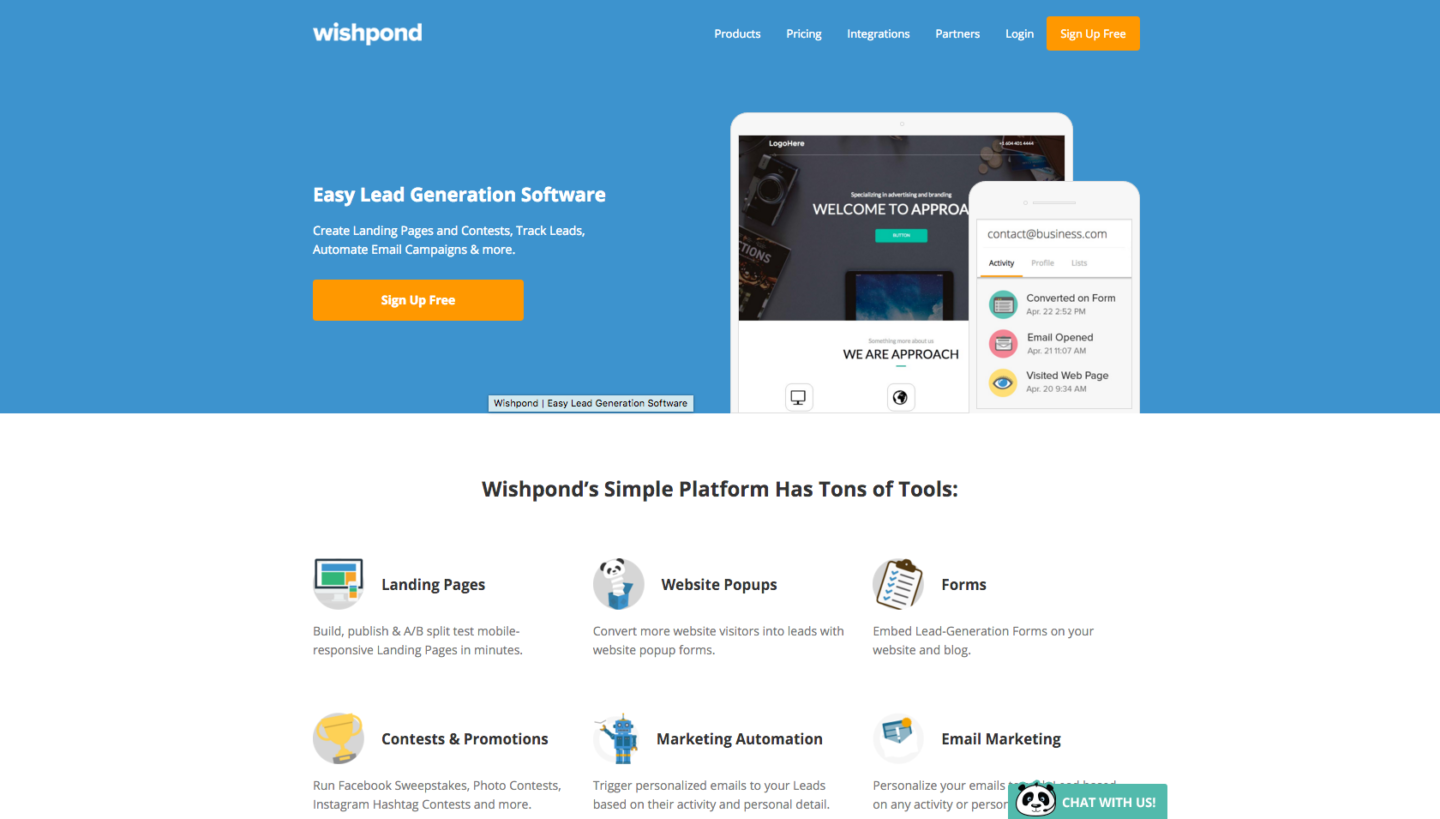Screenshot of the Wishpond Homepage

The top of the Wishpond homepage features a blue background with the brand name "wishpond" prominently displayed in lowercase letters. To the right of the logo, navigation options are available: "Products," "Pricing," "Integrations," "Partners," "Login," and a "Sign Up Free" button.

Below this, in a clean and concise format, the text reads: "Easy lead generation software. Complete landing pages and contests, track leads, automate email campaigns, and more." Another "Sign Up Free" button is located here for ease of access.

To the right of the introductory text, there's an image of a phone screen displaying cropped information. It shows a partially visible message, "welcome to a pro," followed by a truncated display of various user interactions:

- Email contact: "contact@business.com"
- Activity options selected
- Actions such as "Converted on form," "Email opened," and "Visited web page," each with corresponding date and time stamps

Below the main section, the functions of Wishpond's simple platform are briefly described, showcasing a variety of tools:

- Landing Pages: "Build, publish, and A/B split test mobile responsive landing pages in minutes."
- Forms: "Embed lead generation forms on your website and blog."
- Contests and Promotions: "Run Facebook sweepstakes, photo contests, Instagram hashtag contests, and more."
  
Additionally, there is a "Chat with us" button for immediate customer support, and details explaining each function of the platform, reaffirming its comprehensive suite of marketing solutions.